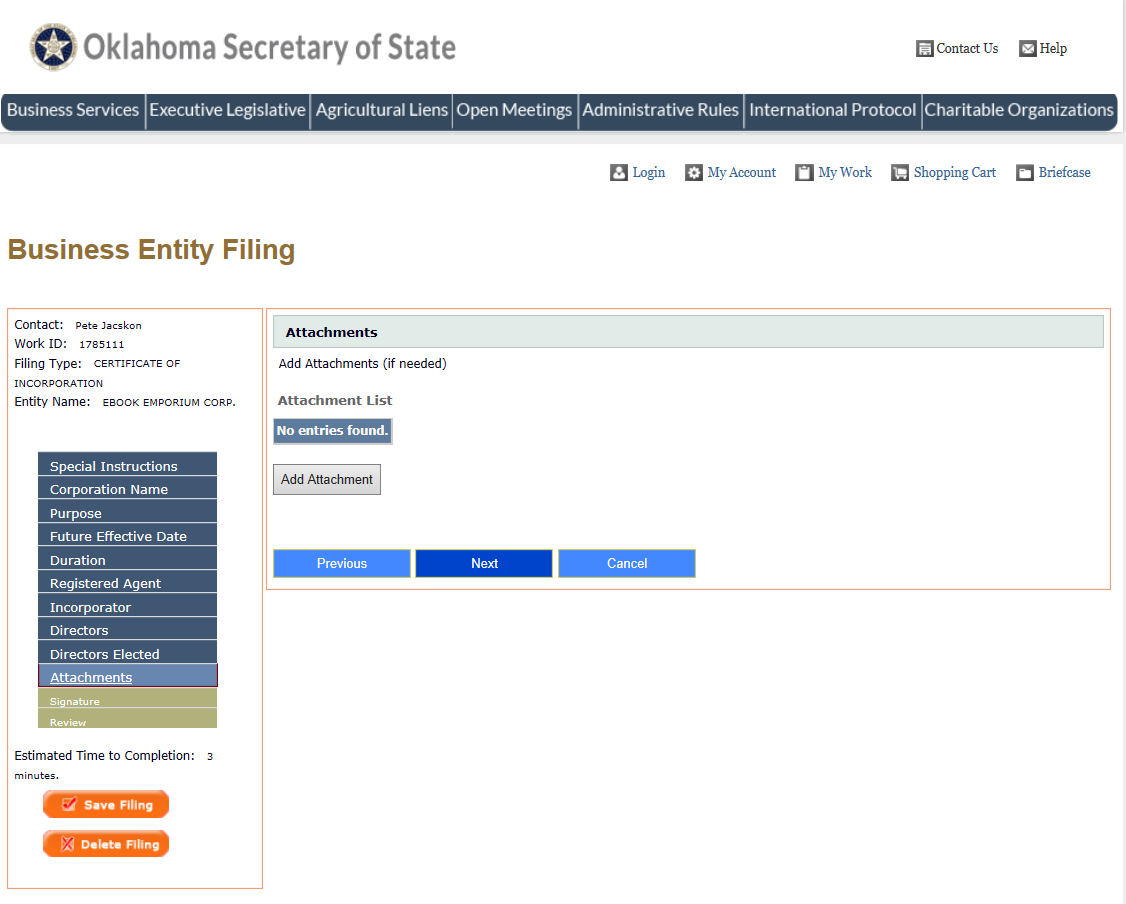The image showcases the Oklahoma Secretary of State's website interface with a highly structured layout. At the top of the page, the header displays "Oklahoma Secretary of State" alongside two links to the right: "Contact Us" and "Help". Directly below this header, there are seven primary navigation categories formatted in blue tabs with white text: 

1. Business Services
2. Executive
3. Legislative
4. Agricultural Lends
5. Open Meetings
6. Administrative Rules
7. International Protocol
8. Charitable Organizations

Beneath the main categories, the website features five user account management options aligned from left to right: 

1. Login
2. My Account
3. My Work
4. Shopping Cart
5. Briefcase

On the left side below these options, there is a section titled "Business Entry Filing" denoted in brown text. This part of the page features multiple tabs, with the top nine being a darker shade of blue, followed by one light blue tab, and two tan-colored tabs below them.

At the bottom of this section, the text "Estimated Time Completion" is displayed. There are two prominent orange buttons: "Save Filing" and "Delete Filing". On the right side of this segment, there is a section for attachments with the instructions, "Add Attachments if Needed" and an indication that no entries are found in the "Attachment Lists". A gray button labeled "Add Attachment" is provided below.

Further below, the navigation includes three buttons: "Previous" in light blue, "Next" in blue, and "Cancel" in light blue. The sections encased in the interface are outlined in orange. The bottommost part of the image displays a white background, prominent in the middle and right-hand side.